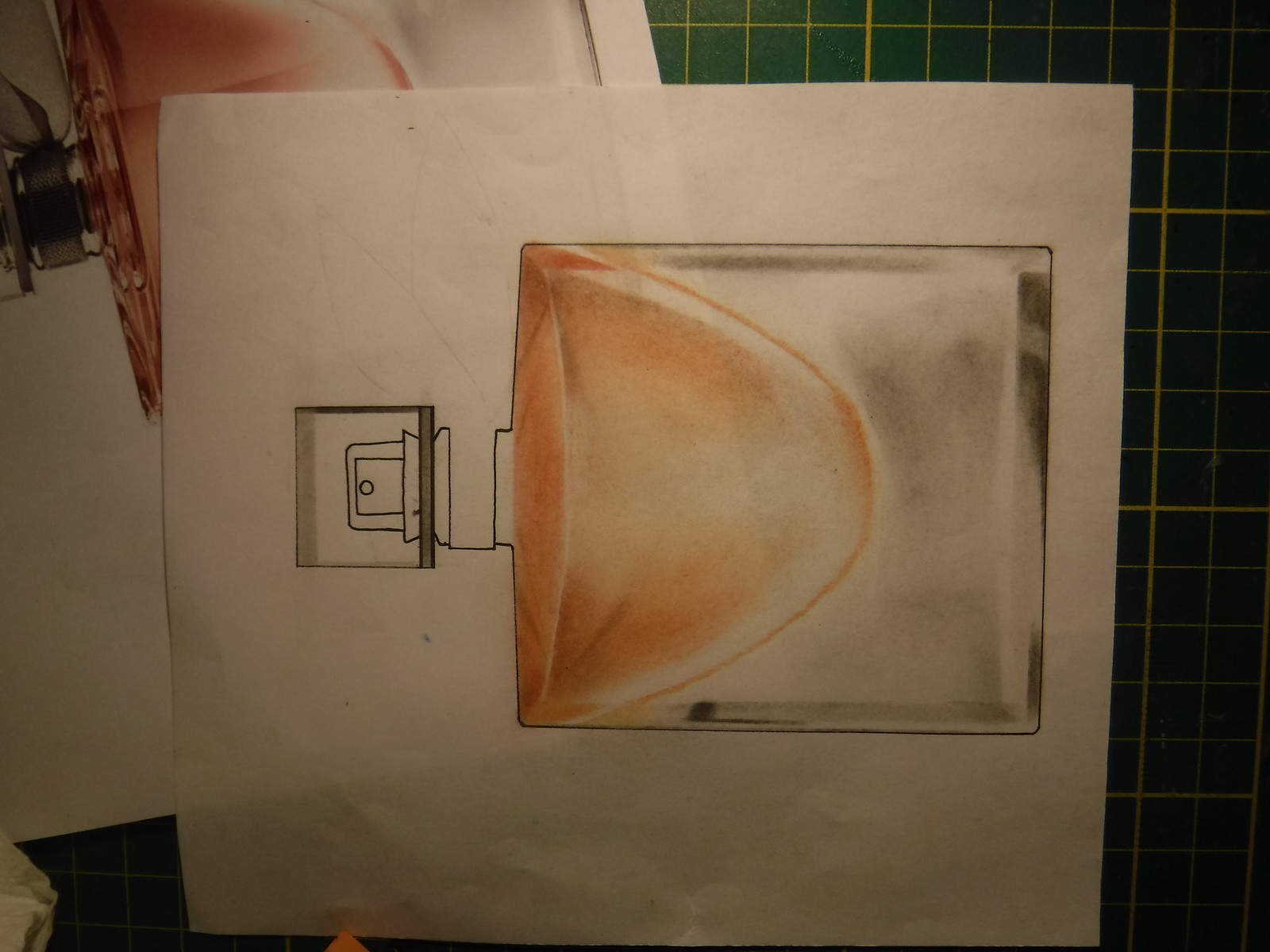A detailed and cleaned-up caption combining the given descriptions:

"This image features a detailed drawing of a perfume bottle prominently displayed on a piece of white paper. The bottle sketch, which is still in progress, showcases a peach-colored liquid filling the bottom half, with the remainder being clear glass and intricate shading details. The unfinished top of the bottle includes an outlined cap and sprayer. Behind the drawing, there is a photograph of the actual perfume bottle, creating a layered effect of concept art over a reference image. Both sheets of paper rest on a green mat resembling a blueprint table, adorned with yellow horizontal and vertical lines. The background mat's pattern, reminiscent of forest green tiles with a dated look and yellow grout, adds a distinctive and structured design to the setting."